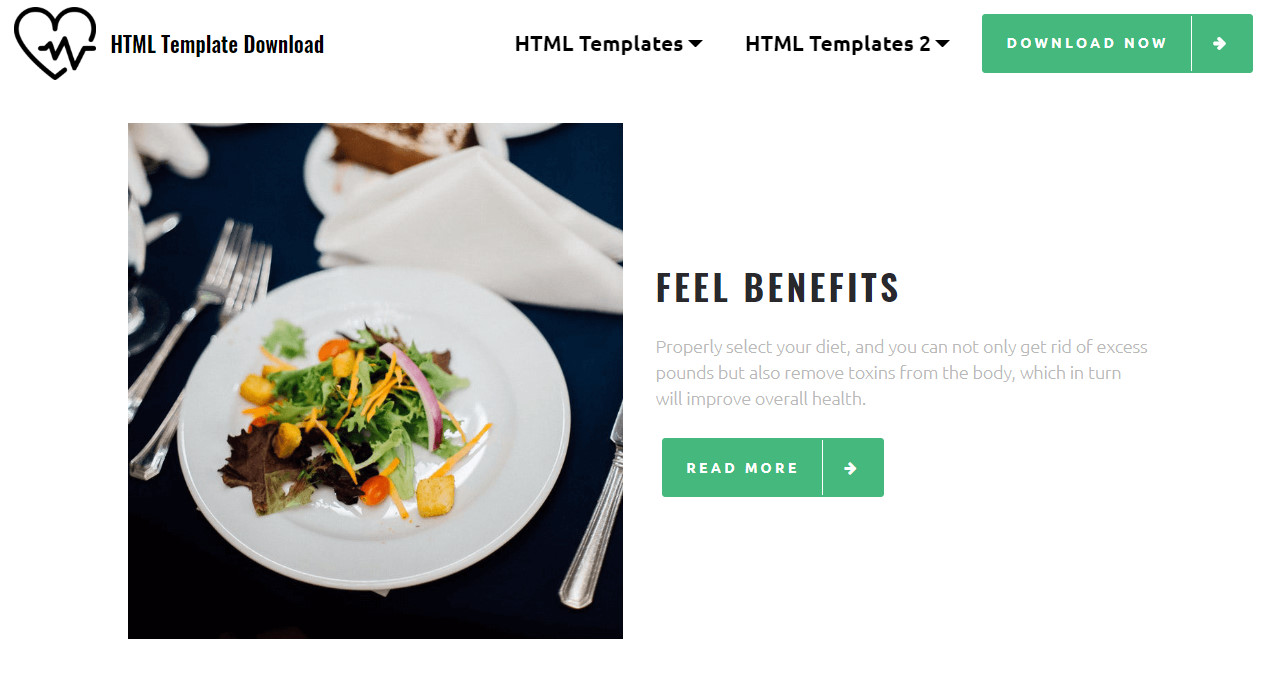The image displays a webpage designed for downloading HTML templates. At the top, there’s a header with a pulsating heart icon beside the text "HTML Template Download." Below it, dropdown menus labeled "HTML Templates" and "HTML Templates 2" indicate different versions available for selection. Adjacent, a prominent green "Download" button stands out.

The main visual element is a white plate with a fresh salad, featuring ingredients like leafy greens, croutons, cheese, onion slices, and cherry tomatoes. The plate is set on a white napkin, flanked by two forks on the left.

To the right of the salad image, text promotes healthy eating with the header "Feel Benefits." The detailed message emphasizes the advantages of a proper diet, including weight loss and detoxification, which contribute to overall health improvement. Below this, another green button invites users to "Read More" about these benefits.

Overall, the webpage combines elements of web design and health promotion, offering users both digital downloads and wellness tips.